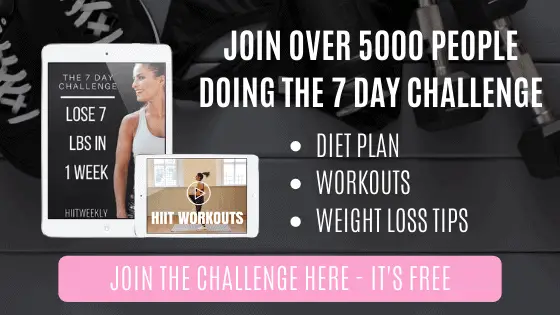Certainly! Here is a detailed and cleaned-up caption for the described image:

---

The advertisement features a striking black background, setting a dramatic tone. Positioned centrally, a pair of black shoes with white laces can be seen, flanked by sleek black and silver weights. Nearby, there is what appears to be a black fabric item, potentially a sports bra or a bag. 

On one side of the image, a simulated tablet screen stands out. The tablet, encased in white, displays a promotion in white text on its black screen: "The 7-Day Challenge: Lose 7 Pounds in One Week." Below this heading, the text "HIIT Weekly" is prominently featured alongside an image of a woman dressed in a white tank top.

Overlaying the central tablet is another white tablet. This second screen shows a woman with a ponytail, poised and ready for her workout. It highlights "HIIT Workouts" as an integral part of the program.

On the opposite side of the image, bold white font reads, "Join over 5,000 people doing the 7-Day Challenge." Below this statement, three white circles list the program's key components: "Diet Plan," "Workouts," and "Weight Loss Tips."

At the bottom of the image, a baby pink rectangular box carries clear white text that entices viewers to "Join the Challenge Here, It's Free." The overall image is crisp with high clarity, and the typography is large and easy to read, making the advertisement both visually appealing and informative.

---